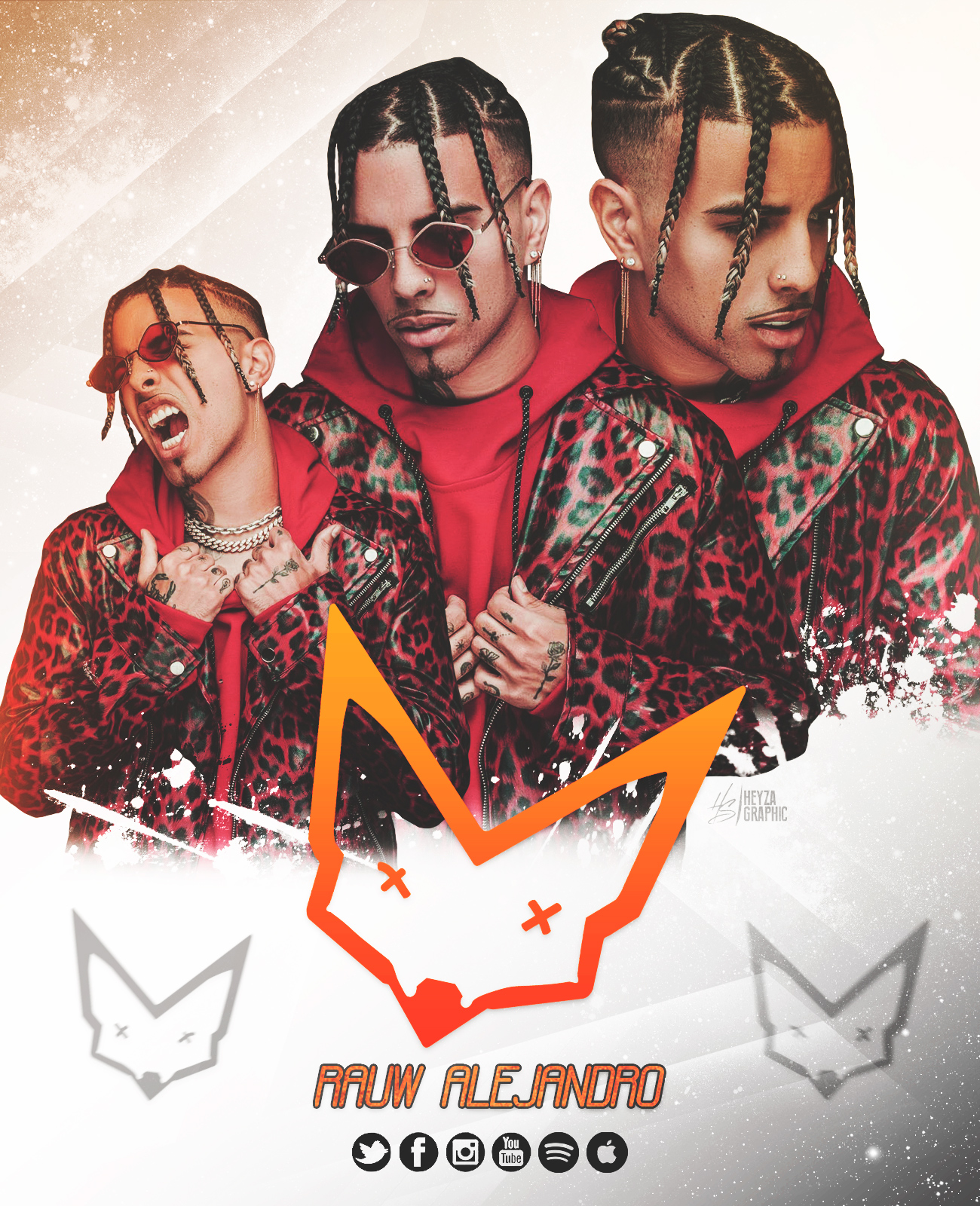This detailed poster features three dynamic images of Ra Alejandro, each showcasing him in a unique pose and expression. In the center of the poster, his stylized sketchy fox logo with X's for eyes is prominently displayed, flanked by smaller, gray iterations on both sides. Above this fox emblem, Ra Alejandro appears in three variations: on the left, he's captured mid-scream wearing red sunglasses; in the middle, he's looking down with sunglasses on; and on the right, he’s gazing to the side without sunglasses. His attire in each image includes a bold red and black cheetah-print leather jacket layered over a black hoodie, along with his distinctive hairstyle of three dreadlocks framing his face.

Beneath his name, “Ra Alejandro,” written in eye-catching orange text with a black outline, the social media icons for Twitter, Facebook, Instagram, YouTube, Spotify, and Apple Music are neatly arranged, indicating where fans can follow his updates and music. Additionally, intricate details like his nose ring, earrings, knuckle tattoos, and neck chains add to his edgy, rebellious aesthetic. The name “Hexagraphic” written in grey text also appears, possibly signifying the designer or production house behind the creative layout. The overall design of the poster serves as an advertisement, highlighting where audiences can connect with and follow Ra Alejandro’s artistic journey.